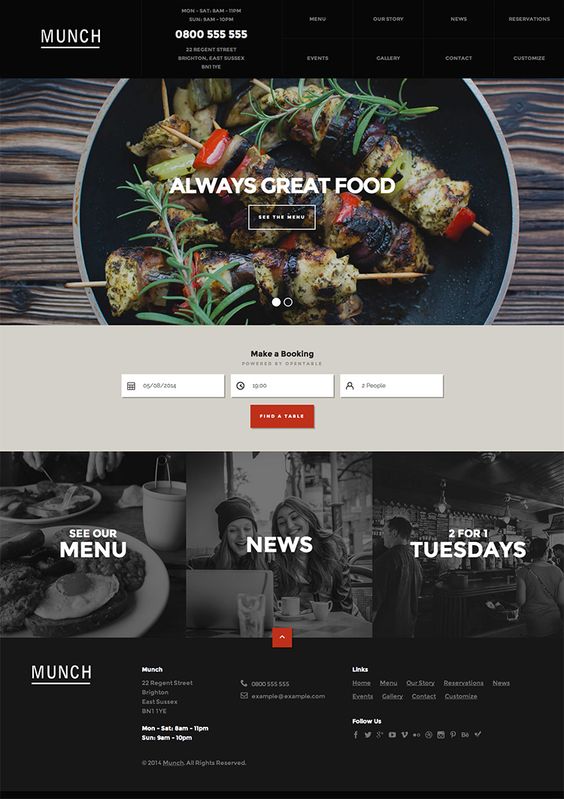The image is a screenshot of a website named "Munch," prominently displayed at the top. The background features a delectable dish, likely shish kebabs, adorned with succulent meat, vibrant peppers, and a sprinkling of fresh herbs, all artfully arranged on a black plate with elegant gold or silver-tinted edges. Above the dish, the phrase "Always Great Food" is inscribed, emphasizing the quality of the culinary experience.

A prominent button labeled "See the Menu" invites users to explore further. Lower down the page, there's a booking section where users can select dates and fill in three fields to find a table. Additional sections at the bottom highlight various offerings, including "See Our Menu," "News," and promotions such as "Two for One Tuesdays."

The top and bottom sections of the website provide navigational links and icons for menu options like "Menu," "Our Story," "News," "Destination," and "Events," offering a comprehensive and engaging user experience.